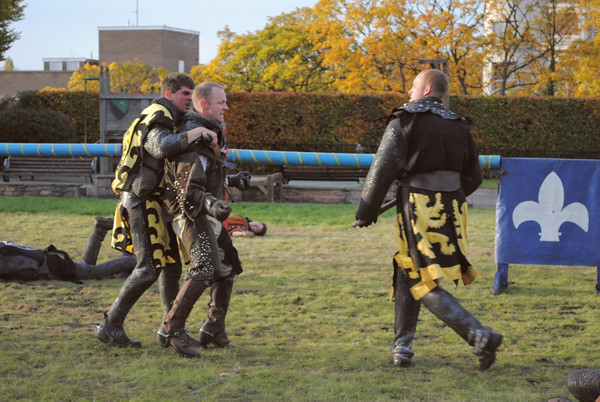In this image, three men are positioned in the center of a flat, grassy field, seemingly recreating a jousting battle. The man on the right is dressed in a black heavy jacket with a short cape adorned with white specks, black cloth wrapped around his waist featuring gold lion insignias, and long black boots. He might be holding a medieval weapon. To his left are two men, one in front and one slightly behind. The man in front, with blonde hair, is dressed in brown boots with silver speckles, brown pants, and a brown jacket. He has his hands clenched in front of him in fists. The man behind him has his arm around his shoulder and is dressed similarly, indicating a shared uniform style.

In the background, there are well-maintained green shrubs followed by trees with yellow and green leaves, suggesting a fall setting. On the far right, a blue banner with a spade shape stands out, and a blue pipe with yellow tape swirling around it stretches from the left to the banner. There are two people lying on the grass, adding to the scene's dynamic nature. Over to the left, a brick building with two levels and a white trim is visible, with an antenna protruding from the roof. The sky is partly visible at the top left, indicating a daytime outdoor setting. The colors in the image include green, brown, black, yellow, blue, and grey, contributing to a vivid and detailed scene.